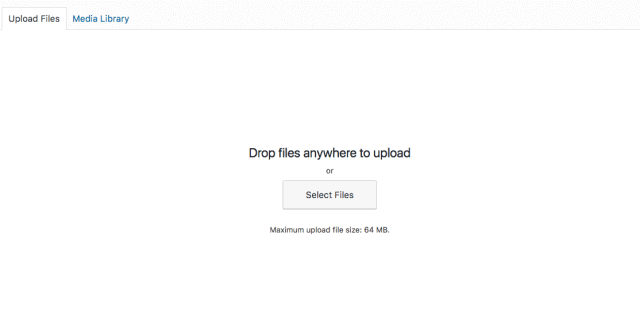The image features a clean, white background with a minimalist design focused on file uploads. At the top of the image, there's a tab navigation bar displaying two options: "Upload Files" and "Media Library," with the "Media Library" tab highlighted in blue, indicating it is currently selected. Just below this, a slim horizontal blue line serves as a separator.

Centrally positioned on the page is a large, inviting text reading "Drop files anywhere to upload," followed by the word "or" which provides an alternative option. Beneath this, a prominent blue button labeled "Select Files" offers users the choice to manually select their files for upload. At the bottom of the image, a small, subtle note informs users that the maximum upload file size is 64 MB. 

The layout is user-friendly, emphasizing ease of use with clear instructions and buttons, facilitating a seamless file uploading experience.